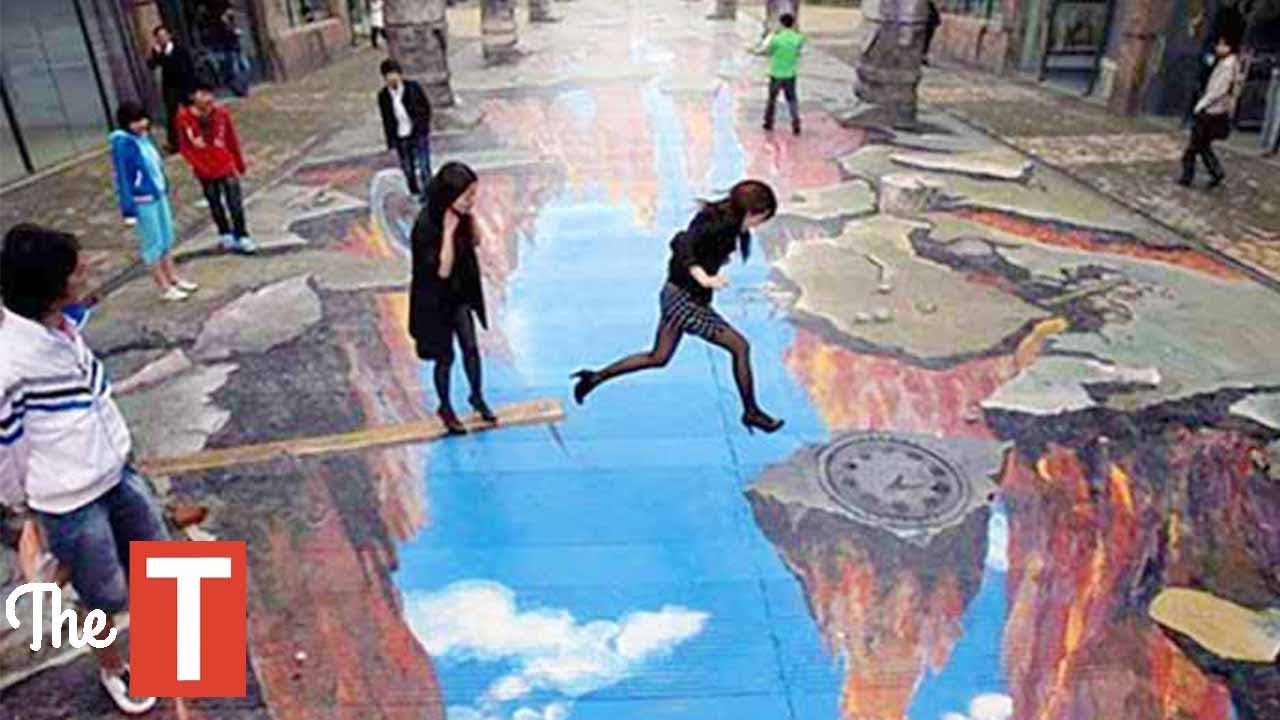The image captures a lively street scene featuring a large, intricate 3D chalk drawing that creates the illusion of a cliff splitting open to reveal a blue sky with white clouds beneath. This stunning artwork spans approximately 20 to 30 feet in width, drawing the viewer's eye from the foreground to the background. On the left side of the street, a young woman stands boldly on a suspended plank that appears to hover over the drawn sky. Midair, another young woman who just jumped off the plank soars above the illusionary abyss. Both women wear black outfits, with one sporting a checkered skirt and high heels. Onlookers line both sides of the sidewalk, marveling at the artwork, while buildings with visible doors and windows, as well as some indistinct large stone structures, frame the scene. In the lower left corner of the image, the word "the" is elegantly written in white cursive next to a prominent red rectangle featuring a capital white "T," suggesting some form of branding or logo.